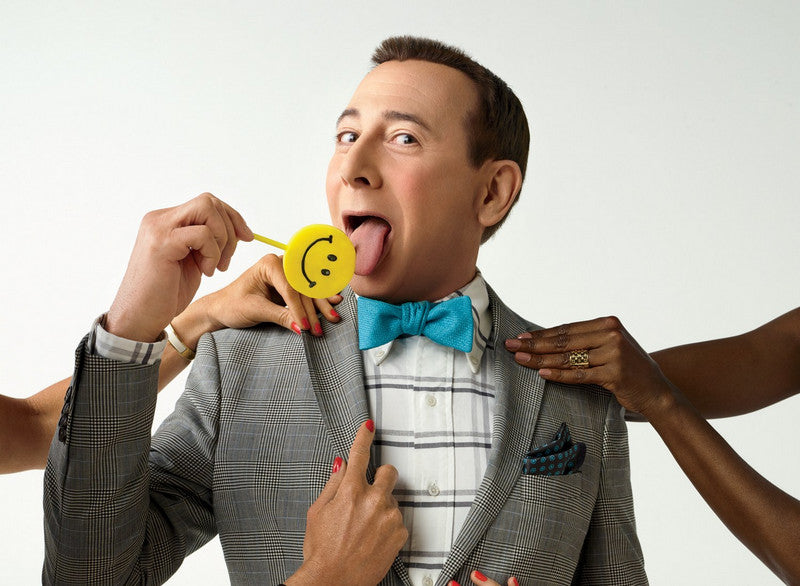This is a color photograph capturing Paul Reubens in his iconic role as Pee-wee Herman, standing at the center of the image in a landscape orientation. He is depicted from the top of his head down to about mid-chest. Pee-wee Herman is wearing his signature gray blazer over a white collared shirt, which features horizontal gray and black stripes, and a light blue bow tie. His right arm is bent at the elbow, pointing a yellow smiley face lollipop towards his mouth. With his mouth open and his tongue extended, he appears to be licking the lollipop while looking slightly to his left. 

Pee-wee is surrounded by several disembodied hands reaching toward him from various directions. Two light-skinned hands come into view from the bottom of the photo, one touching his right lapel with red-painted fingernails on the thumb and forefinger, and the other showing just the tips of a couple of fingers with similar red polish. A dark-skinned hand, wearing a ring on the ring finger, extends from the right edge of the photo to rest on his left shoulder. Another light-skinned hand with red-painted nails is visible on his right shoulder, emerging from the bottom left corner of the image. Pee-wee’s playful expression and the whimsical elements of the scene, combined with the hands reaching towards him, create a distinctive and surreal vibe. The background of the image is solid white, allowing Pee-wee and the intruding hands to stand out prominently.